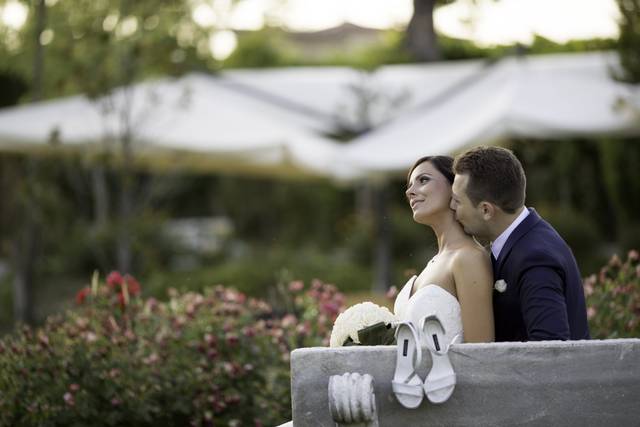In this photographic image taken outdoors during the early evening, a bride and groom are seated on a wooden bench, positioned sideways to the camera. The bride, in a white, strapless wedding dress with a sweetheart neckline, has her brown hair pulled back and is holding a bouquet of white flowers. She is smiling gently and looking up with her head tilted as the groom, who has short brown hair and is dressed in a navy blue suit with a white shirt and a flower in his lapel, kisses her neck from behind. Her white sandals dangle from the top of the bench, adding a casual yet intimate touch to the scene. The background is slightly out of focus, featuring a mix of red and purple flowers on green bushes, a series of tents suggesting a wedding reception, and a blend of green trees against a twilight sky that transitions into a pale white-orange.